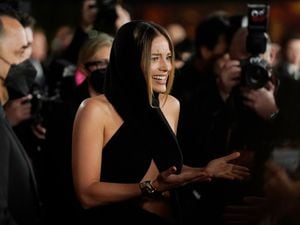In the image, a familiar-looking actress with shoulder-length dark brown hair, lighter at the ends, is at the center of attention. She is dressed in a striking black dress with criss-cross straps creating a keyhole opening at her stomach and extending up around her neck. Her pose, with both arms bent at the elbows and palms facing up, complements her surprised and joyous expression, as if she has just won an award. The scene is bustling with photographers capturing her reaction, while some onlookers and a couple of masked individuals, including a man who might be a bodyguard and a woman in glasses, observe the moment. The actress's apparent delight amidst the flurry of camera flashes creates a dynamic and celebratory atmosphere.